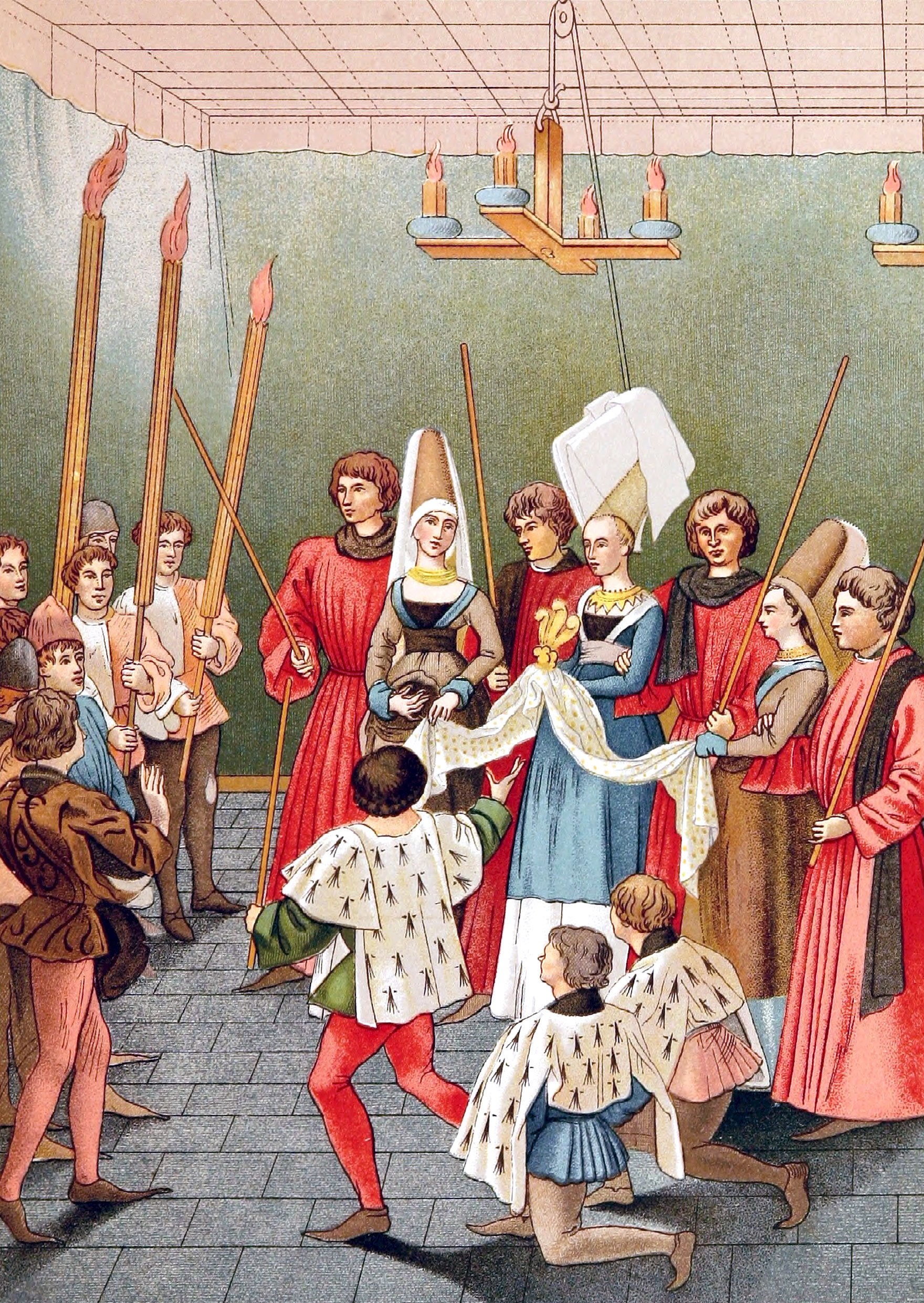This rectangular artwork depicts a historical scene featuring a group of people indoors. At the center of the image, a woman who appears to be of royalty is prominently positioned. She is adorned in a blue and white dress, a tall white fabric headpiece, and a gold piece around her neck, while the white scarf in front of her bears a crown design. Flanking her are men wearing long red gowns, suggestive of the old-fashioned attire once associated with nobility. The left side of the image shows a different group of people dressed in more casual brown and tan colors. These individuals are holding torches with orange flames at the tips. Two people can be seen kneeling near the center, further indicating the presence of royalty. The background of the scene features a green wall and a pink ceiling, with candles hanging from a chandelier on a pulley system above. The ground is constructed of gray stone in a square or rectangular pattern.